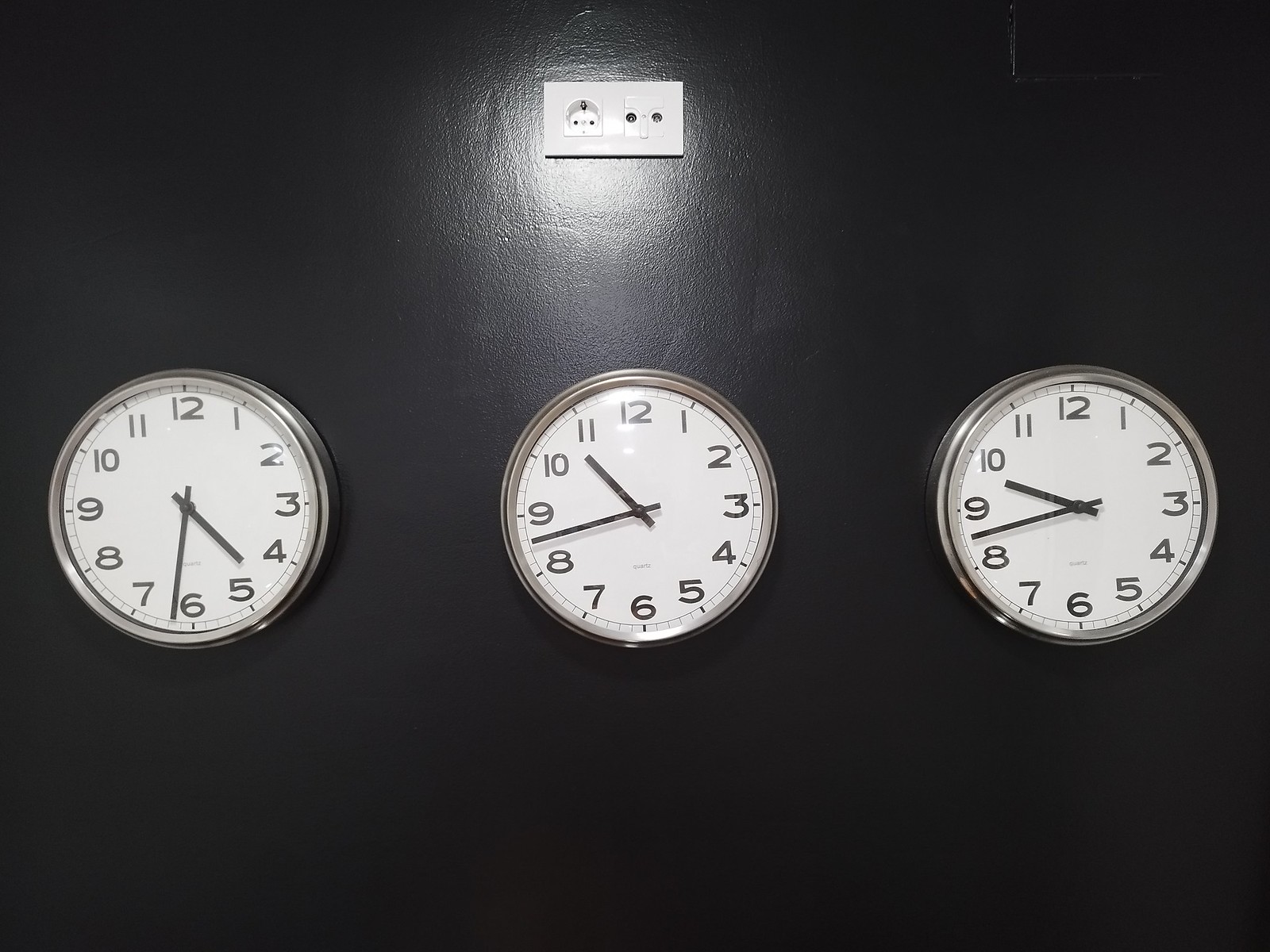The image depicts a sleek black wall featuring three traditional analog clocks in a minimalist design, each with a black and white color scheme and standard clock hands. Positioned above the clocks are what appear to be wall outlets, though their purpose is unclear. Focusing on the time displayed by each clock, the clock on the left shows the hour hand slightly past 4 and the minute hand at 6:10. The middle clock's hour hand is just before 11, with the minute hand indicating 8:30. On the right, the clock's hour hand is a little before 10, while the minute hand also reads 8:30.